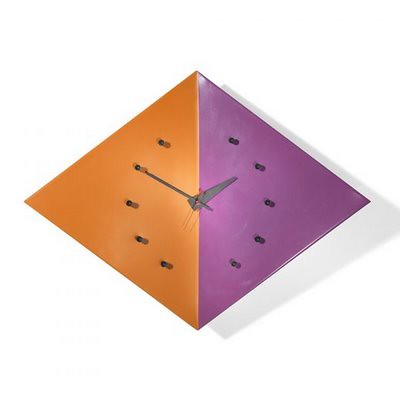This image depicts a three-dimensional clock, isolated against a transparent background. The clock's design suggests a geometric structure with four visible sides and a base likely forming a square. The clock face features two prominent triangular sections: an orange triangle on the left side and a purple triangle on the right. 

The clock lacks any numerals; instead, it employs metal hands in the center to indicate time, comprising a minute hand and an hour hand. Surrounding the clock face are small dots marking the hours. The orange triangle contains five dots, and the purple triangle mirrors this with an additional five dots, resulting in a total of ten dots marking the hours between them. The position for the 12th hour is notably absent. The overall design of the clock is modern and minimalist, with a clear focus on geometric shapes and simple, clean lines.